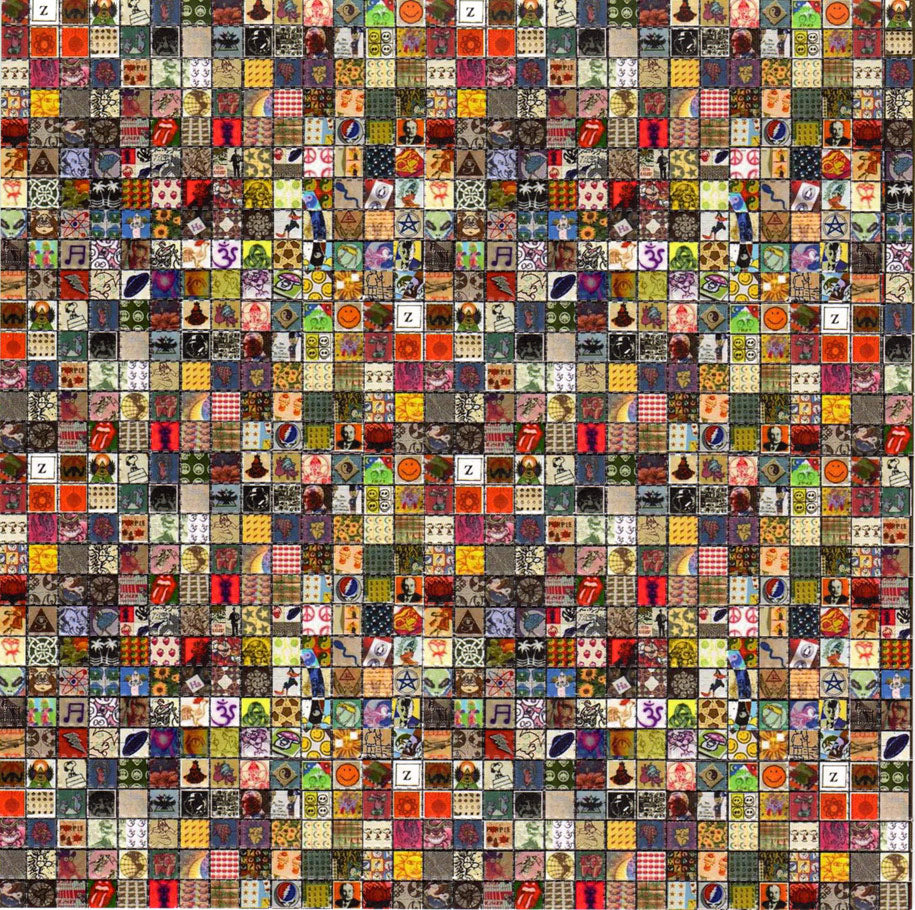This image is a digital mosaic or quilt composed of a 28 by 28 grid, resulting in 784 individual tiles. Each tile features a unique or repeated, recognizable image. Among the numerous small tiles, repeated logos and symbols can be identified: the iconic red lips with a tongue sticking out, reminiscent of the Rolling Stones band logo; an orange smiley face; and the distinctive red, white, and blue Pepsi logo against a gray background. Additional elements include green alien heads, illustrations of sunflowers, yellow tiles with sun illustrations, a Pink Panther logo, a soccer ball with beige and brown patterns, an image of Buddha, Arabic symbols, peace signs, and even a small illustration of a sperm cell. This intricate, colorful grid highlights the variety and repetition of popular symbols and images.